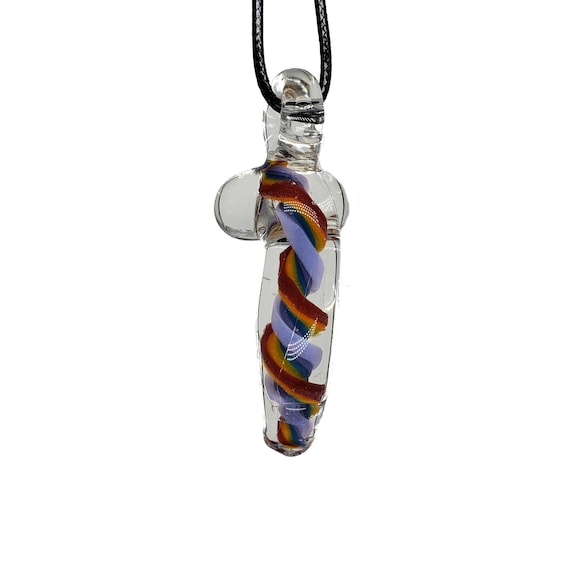The image showcases a long, circular glass instrument hanging from a black cord, centrally positioned. The glass object is intricately see-through, revealing two spiraled materials within. One spiral exhibits a vibrant array of red, yellow, and green colors, while the other displays a combination of blue and purple hues. These spirals twist and interlace as they descend through the interior of the glass structure. The object itself is an elongated tube that slightly bulges out, forming a rounded hook at the top where it is suspended from the black cord. The exact purpose of this decorative, rainbow-hued device remains unknown.